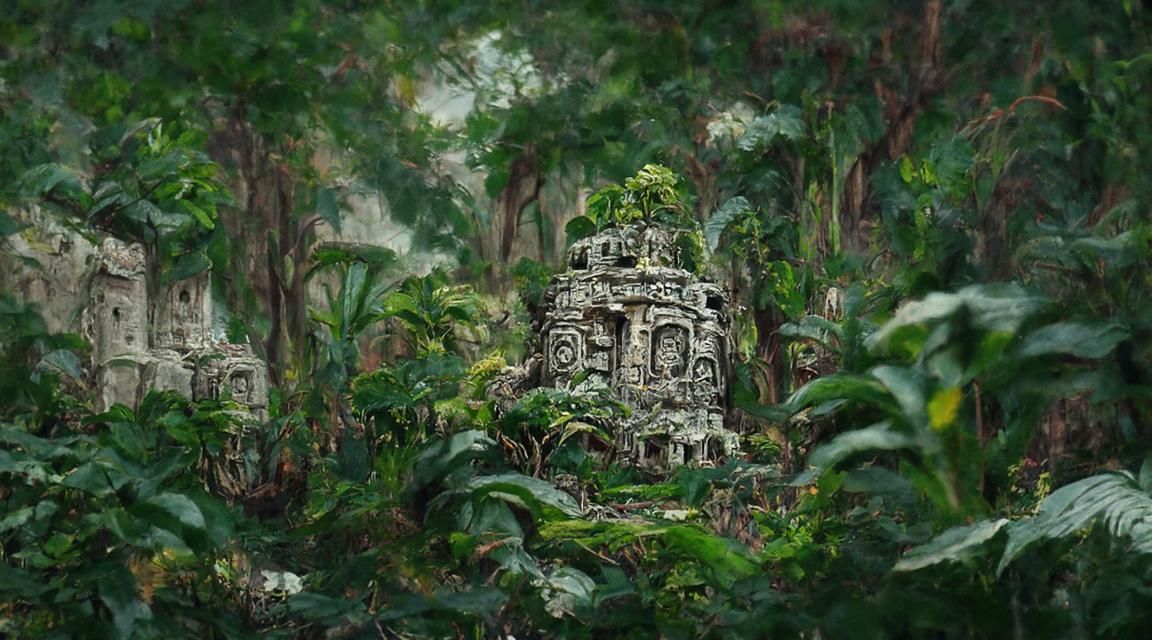In a horizontally aligned rectangular image reminiscent of a video game scene, the lush, deep green forest creates an immersive backdrop that appears almost miniature and AI-generated. The image evokes a blend of realism and an artistic touch, particularly at the blurred, smudged edges, giving it a painted appearance. The scene, rich in greens, yellows, and browns, is dominated by dense vegetation—large, overgrown leaves and grasses fill the foreground, providing a vivid and lifelike texture.

At the center and left side of the image, two prominent stone structures emerge from the foliage, partially obscured by the dense jungle. These ancient ruins are crafted from aged, concrete-like material, reminiscent of Mayan and Aztec architecture. The larger, cylindrical structure in the center is ornate, featuring intricate designs, while the square, rock-like formation to the left stands robust and irregular. Both structures suggest ancient, overgrown buildings or castles hidden away in a lost South American jungle.

The tops of the trees in the background blur into the cloudy, gray sky, barely visible through the thick canopy. The subtle hues of brown bark and stems interspersed amongst the green add depth to this intricate scene, enhancing the mysterious allure of these ancient, forgotten runes enveloped by nature.